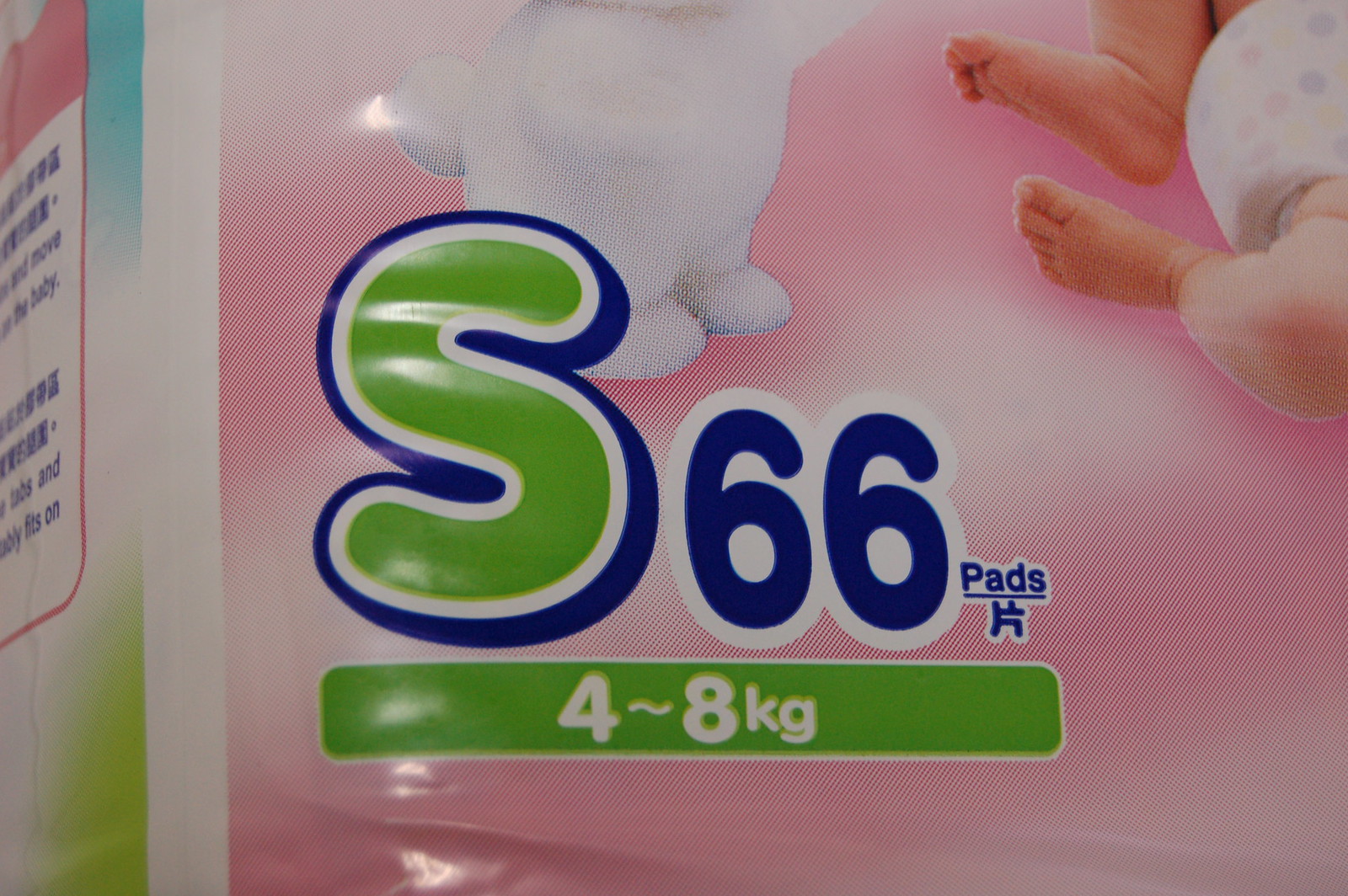The image is a very close-up view of a package, likely for baby diapers or diaper liners, from a different country, with text and labels possibly in Chinese. The pink background features fluffy white clouds and a round-bodied, white, fluffy-tailed creature, probably a bunny, prominently displayed on either the front or side. In the top right corner, a baby's feet, wearing a lavender and pink polka-dotted disposable diaper, can be seen. Central to the image is a large green 'S', outlined in white and blue, next to a blue '66' also outlined in white. Below, a long green rectangle contains the text "4 to 8 kilograms" in white. The word "pads" appears in small blue lettering, outlined in white, below the '66'. On the left, part of a possible warning label with Asian characters is visible.